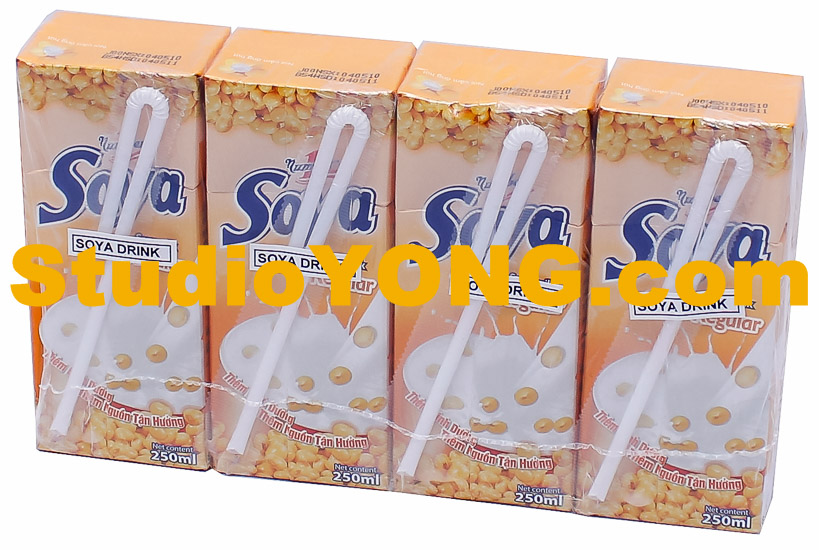The image showcases four light tan, rectangular drink boxes labeled "Sala" or "Soya," each adorned with a bent white straw taped to the front. These containers, reminiscent of juice boxes, are possibly cereal-based drinks, as they feature imagery of cereal and milk. The boxes, which appear to be saran-wrapped together, have orange writing and a peach-colored design. The words "studioyoung.com" are prominently displayed in front of the drinks, indicating a contact or brand website. The backdrop of the photograph is completely white, making the details of the packaging and the promotional information stand out clearly. Each box also has a small foil spot where the straw can be inserted for drinking.